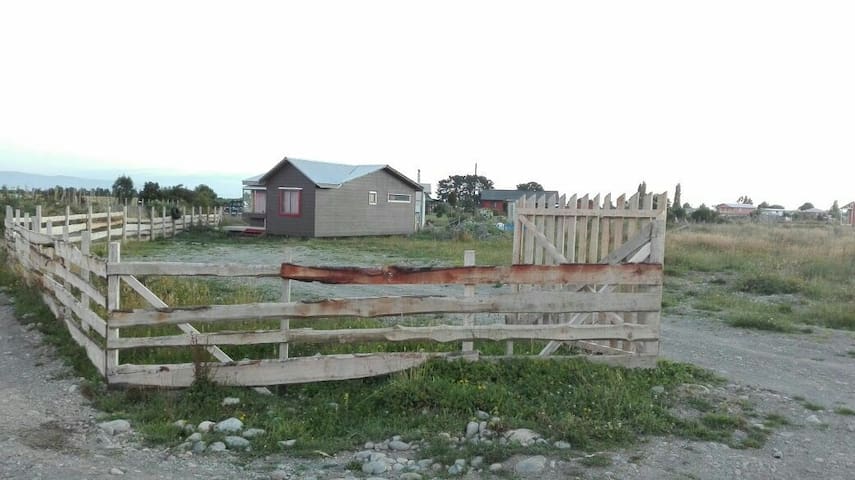This picture captures a rural scene with a weathered, rickety wooden fence that prominently spans across the foreground, showcasing significant deterioration, potentially from fire or rot. The fence, light brown in color and full of gaps, encloses a property featuring an old, single-story house with a light gray roof. The house, modest and plain, sits centrally in the image with the right-hand side showing an open gate leading to a dirt driveway. The fence appears to wrap around the property, highlighted by patches where it seems considerably more damaged. Surrounding the fence is a rough mix of gravel, dirt, rocks, and sparse grass. In the background, faint outlines of distant houses and mountains can be seen, though much of the background blends into a nearly white, almost transparent sky, contributing to an eerie sense of isolation. The driveway, albeit indistinct, stretches from the gate to the lower right corner of the image, merging with grass and dirt, further enhancing the scene's desolate and unkempt appearance.